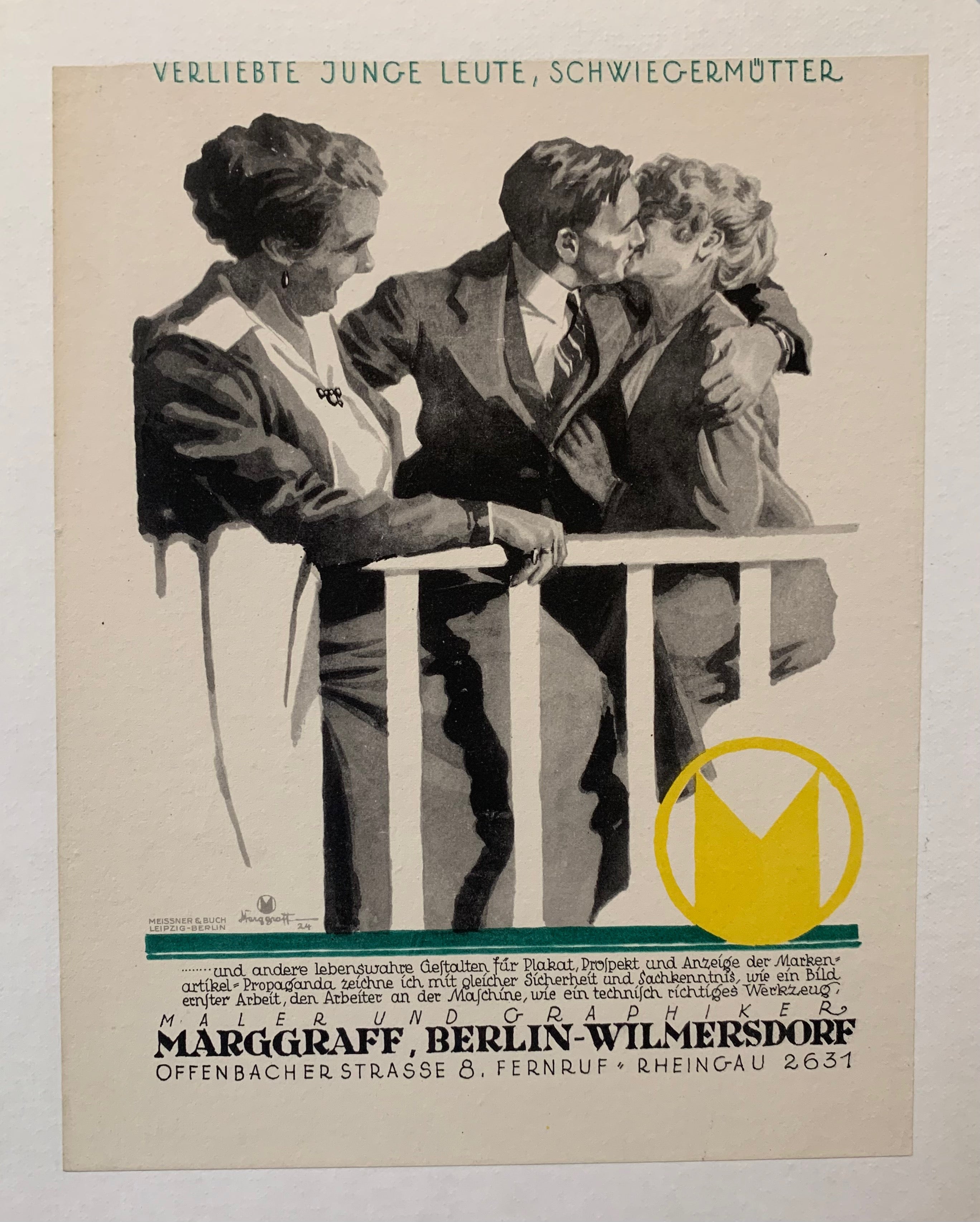This is an intricate black and white drawing featuring German text. At the center, a scene unfolds on what appears to be a balcony with a white railing. A woman, dressed in a 1930s-style business suit, is leaning against the railing, smiling warmly. She observes a man in a suit, complete with a white shirt and striped tie, as he kisses a blonde-haired woman seated in a dress. The image is distinctly from an earlier era, evoking the elegance of the time. Beneath the illustration, the text reads: "Mähler und Grafinger" with additional annotations: "Margrath of Berlin, Wilmersdorf, Offenbacherstrasse, 8, Fernroth, Rheingau 2631." Though the exact meaning of the German text remains unclear, it adds an authentic historical and cultural context to the scene.